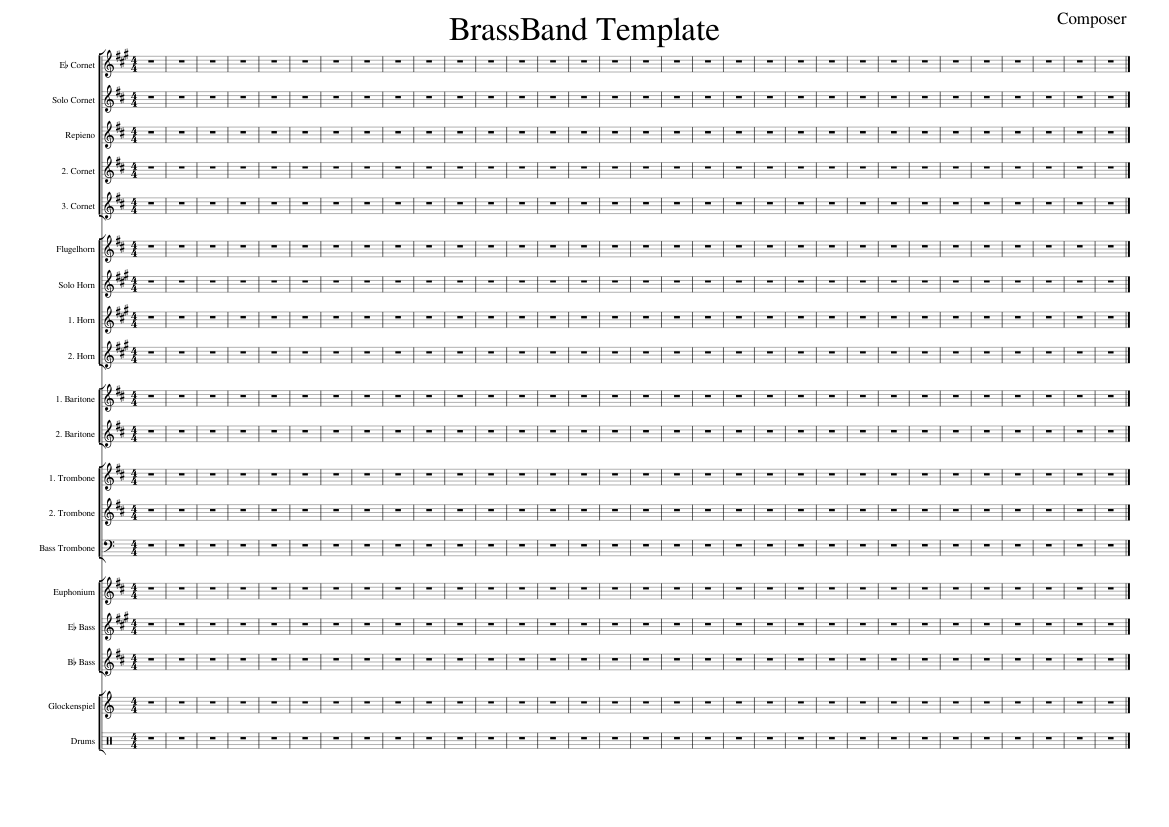The image depicts a black and white template for writing a musical score, specifically titled "Brass Band Template" prominently displayed at the top center. On the far right of the top margin, the word "Composer" is printed. The page is filled with rows of musical staves, each adorned with a treble clef symbol on the far left. Instead of traditional notes, a repeated dashed line is centered on each staff. Along the left margin, there is a vertical column listing instrumental parts like "EB," "Cornet," "Solo Cornet," and "Fugle Horns," but no actual music is written out. The clustered musical symbols at the start of each line, presumed to be the staff notation, emphasize the template nature of this sheet music, awaiting composition. Toward the end of each row, the lines visually thicken, suggesting a section yet to be annotated.